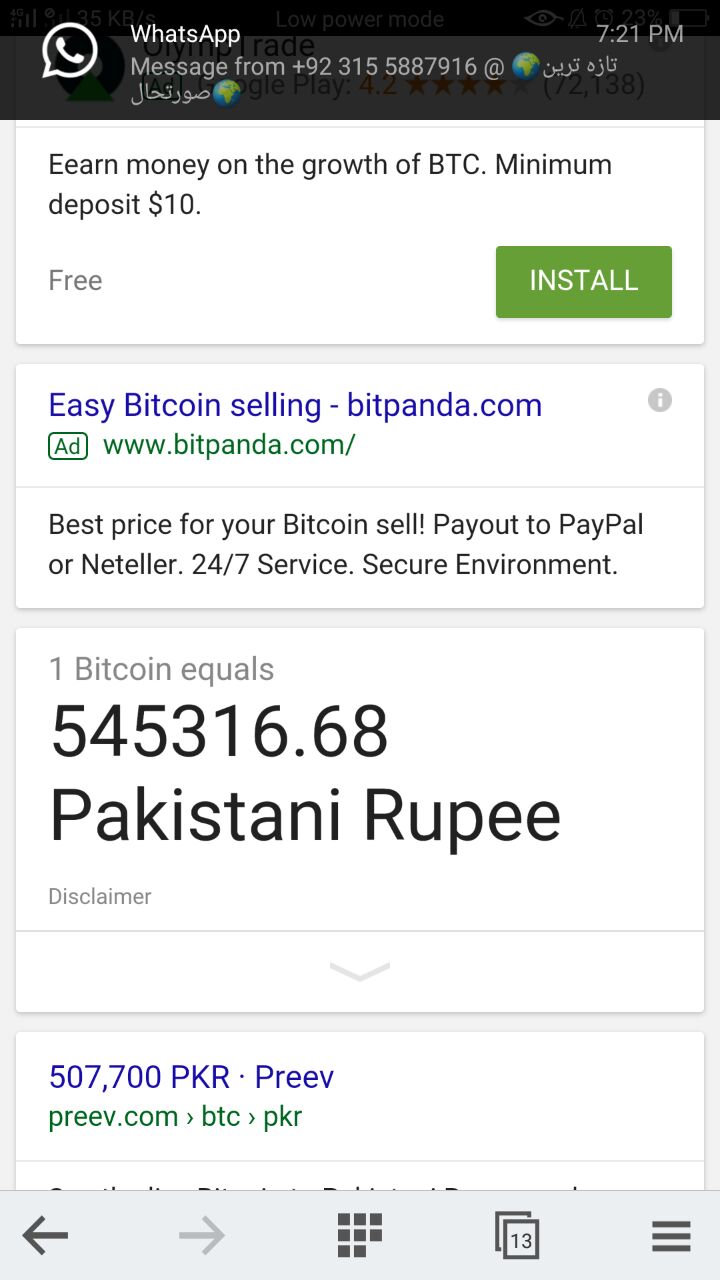This detailed caption describes an image of a WhatsApp page with various elements related to Bitcoin trading and information:

---

The image depicts a screenshot of a WhatsApp page, identifiable by the black header at the top that reads "WhatsApp." Displayed at 7:21 PM, the message originates from an international number. At the top, there is a white message icon with a phone inside it. 

The message reads: "Earn money on the growth of BTC. Minimum deposit $10." The word "Earn" is initially misspelled as "Eearn." The text includes a green button with the white lettering "Install." 

Below this section, there is information about Bitcoin selling, directing users to visit "bitpanda.com" for the best prices. It states: "Best price for your Bitcoin. Sell, payout to PayPal or Neteller. 24/7 service. Secure environment.”

Further down, the image displays the current exchange rate for Bitcoin: "1 Bitcoin equals 545,316.68 Pakistani Rupee." A disclaimer is noted below this information. 

There is also a drop-down button visible. The subsequent line lists another exchange rate: "1 Bitcoin = 507,700 PKR," sourced from "preev.com."

Overall, the image provides detailed information regarding Bitcoin trading options, exchange rates, and services within a WhatsApp message format.